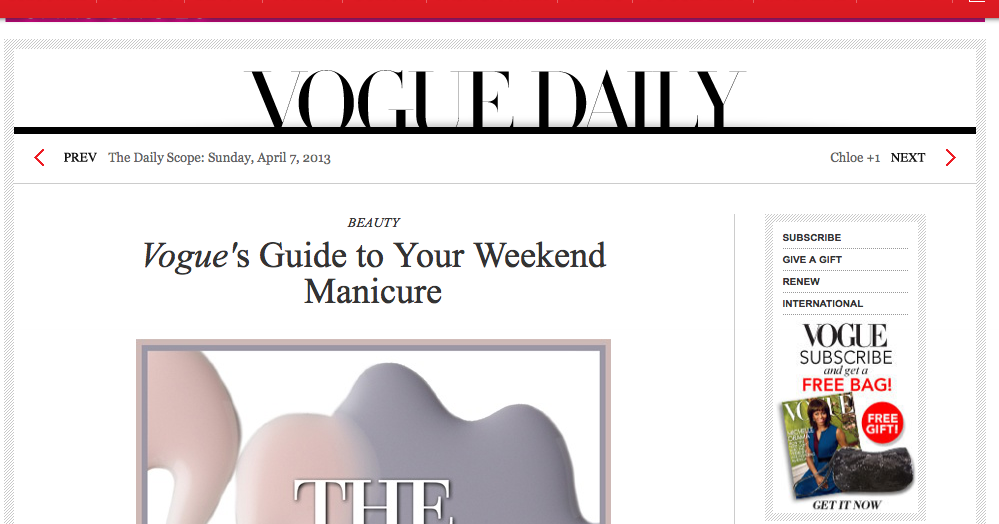The image is a snippet of the cover of Vogue magazine's blog or website, characterized by distinctive design elements and informative content. At the top, there is a red banner bar with a shadow effect, suggesting a deep maroon-purple hue. Following this, a section of white space leads to the main content outline, which is rendered in a light, transparent gray.

Prominently displayed just below is the title "VOGUE DAILY" in all caps, underlined by a dark line stretching across the width of the section. Beneath this, text reads "PREVE LIKE PREVIOUS" followed by "THE DAILY SCOPE, SUNDAY, APRIL 7, 2013." To the far right, "CHLOE PLUS ONE" appears in gray, followed by the word "NEXT" in bold black uppercase letters, accompanied by a red arrow.

As you scroll down, the headline of the first featured article from the beauty section is introduced in italics with "VOGUE," followed by "GUIDE TO YOUR WEEKEND MANICURE" in non-italicized text. The introduction to an article on nail polish follows. To the right of the main content, options to "SUBSCRIBE," "GIVE A GIFT," "RENEW" and more are available, providing readers with various actions to engage further with the magazine.